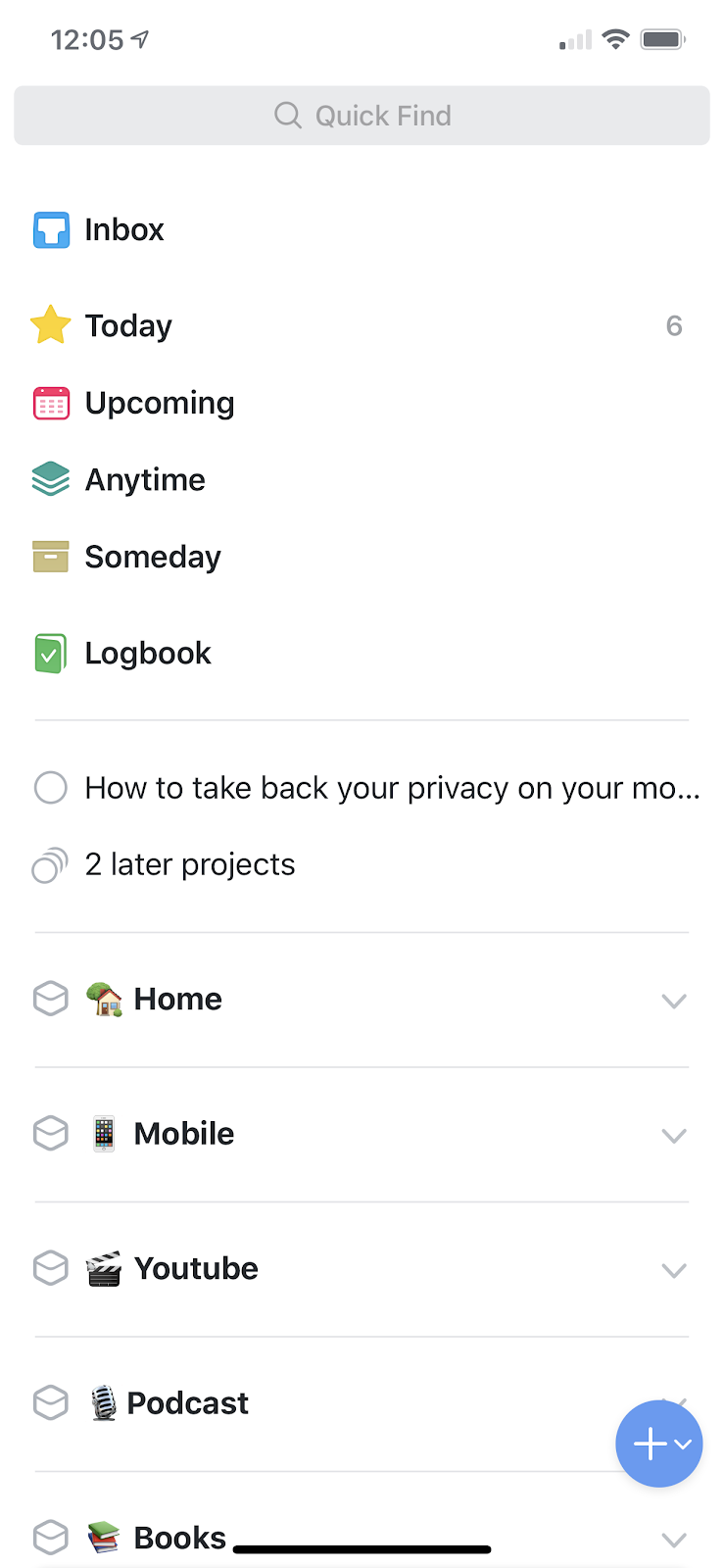The image displays a screenshot from a cell phone. In the upper left corner, the time "12:05" is shown in gray text. The upper right corner indicates one bar of cellular reception, Wi-Fi is enabled, and the battery icon is full. Just below the status bar, in light gray text, the phrase "Quick Find" is displayed.

The interface includes several categories listed vertically: "Inbox," marked with a star next to "Today," a small calendar icon next to "Upcoming," followed by "Anytime," "Someday," and "Logbook." These categories are separated by a very light gray horizontal line.

Below this line, there is a partially visible text reading "how to take back your privacy on your" and "later projects." Further down, various icons and their corresponding labels are listed: a house icon with "Home," a cell phone icon with "Mobile," a movie screen icon with "YouTube," a speaker icon with "Podcast," and at the bottom, an icon of books labeled "Books."